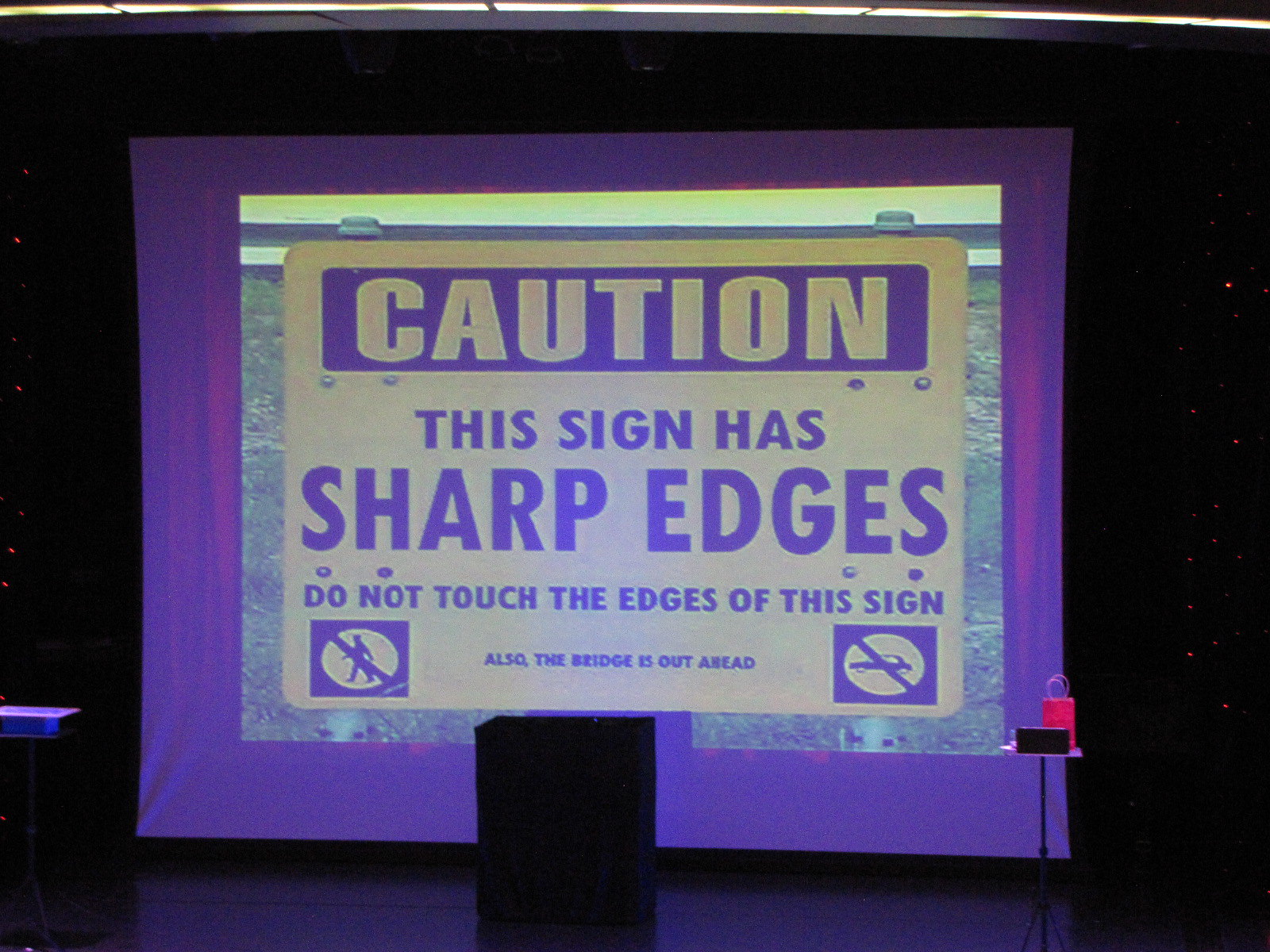This indoor photograph captures a stage setup during an ongoing presentation, prominently featuring a humorous caution sign projected onto a white screen. The screen is visible amidst a dark backdrop and a few small red dots. Centered on the screen, the yellow rectangular sign warns, "Caution! This sign has sharp edges. Do not touch the edges of this sign," although the sign's edges are actually rounded. The caution is flanked by a crossed-out image of a walking person on the bottom left and a car on the bottom right, with additional text noting, "Also, the bridge is out ahead." The stage layout includes a dark-colored podium in the center, a small table with a black box and a pink party gift bag to the right of the screen, and another table situated at the bottom left.